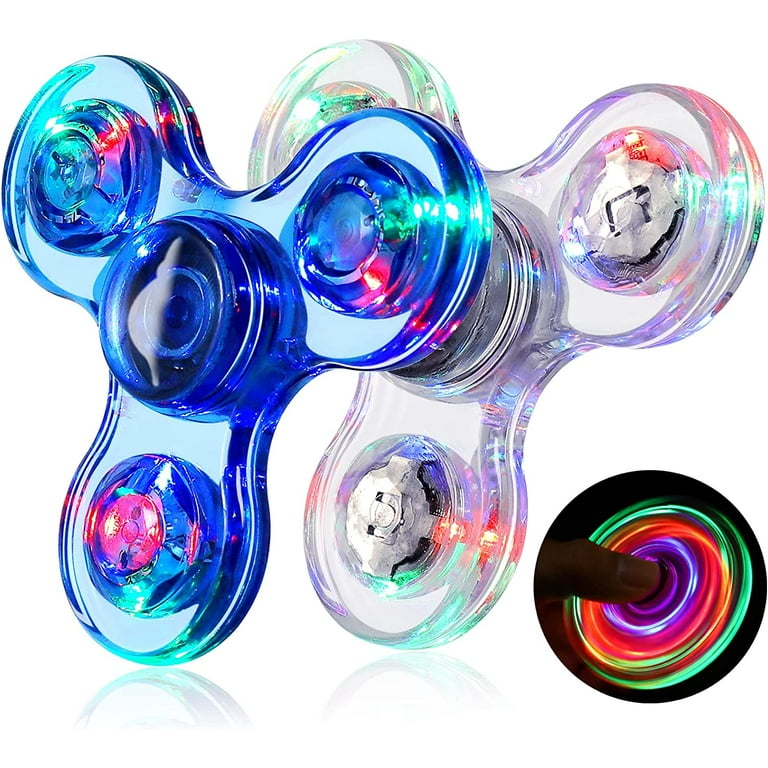This product photograph, typically used for commercial listings on online websites or catalogs, features two fidget spinners positioned against a flat white background. The fidget spinners, renowned for their popularity about a decade ago, are stacked one on top of the other. Each spinner is structured with a central circular hub connected to three circular lobes, designed for ease of spinning between fingers.

The top fidget spinner is a semi-transparent blue, while the one underneath is clear and fully see-through. Both spinners are made from a semi-see-through plastic material. Embedded within each of the three peripheral circles of both spinners are small batteries and dual LED lights, which can illuminate in green or red. The specified design includes a clear depiction of the LED lights when activated, creating a vibrant display of colors during use, though the image itself doesn't show the lights in motion. In addition, the structured sections contain intricate designs or faces that are not detailed enough to identify but add to the visual intrigue of the spinners. This detailed image highlights the aesthetic and functional features of these classic toys, emphasizing their nostalgia and appeal in a modern, polished presentation.